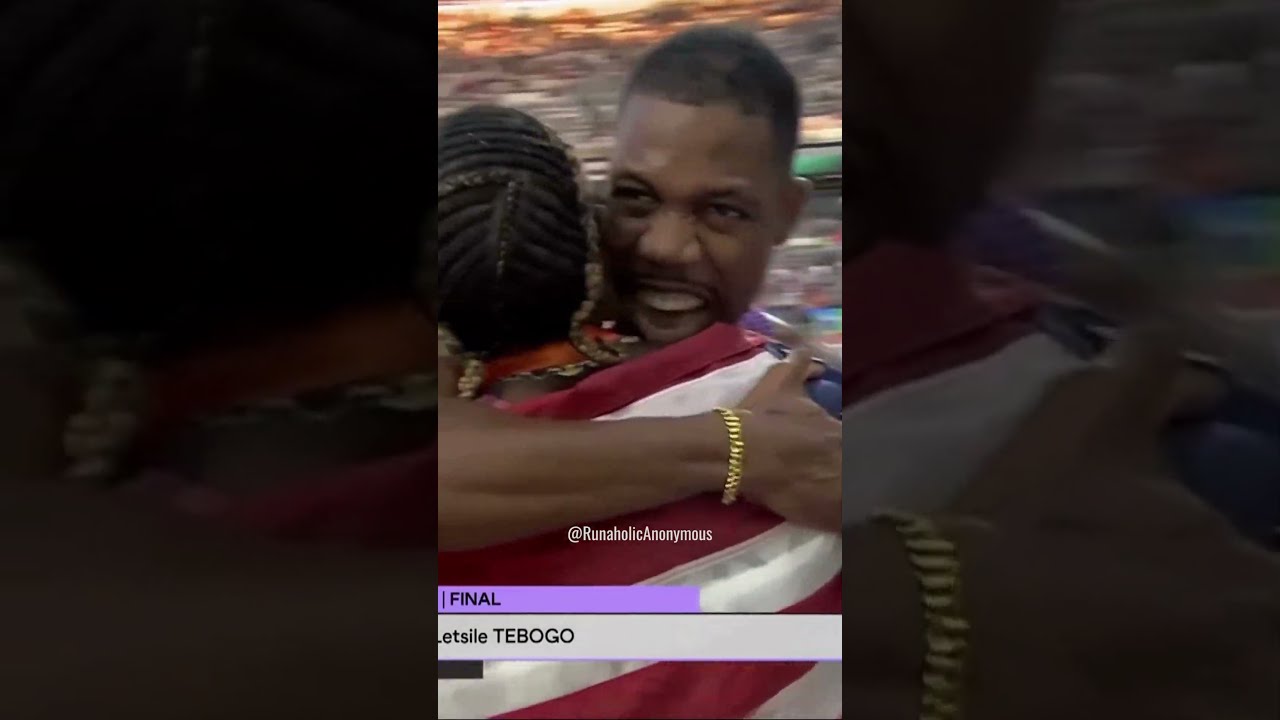This horizontal rectangular image prominently features a joyous embrace between a man and a woman in the center, with the sides of the picture blurred, hinting at a close-up shot. The man, an African-American with short black hair and a thin mustache, has his mouth wide open in a delighted laugh, revealing his teeth. His arm, adorned with a gold bracelet, wraps around the woman's back. The woman, who could potentially be a little girl, also appears to be African-American with tightly braided black hair interspersed with longer light brown braids, and dons a horizontally striped jacket of alternating red and white stripes. The scene hints at an emotional moment, possibly at a sporting event, inferred from the dense, two-tier bleacher of blurry audience members in the background, suggesting a large crowd. An American flag is draped over the woman's shoulder, and the text "@Runaholic Anonymous" is visible slightly below the middle of the image, with the additional words "final" and "Tebogo" at the very bottom.